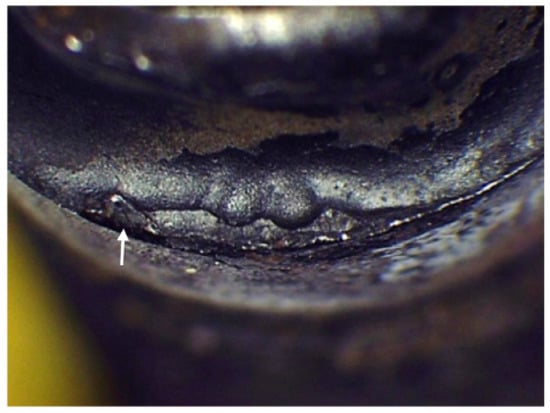The photograph, rectangular and oriented horizontally, remains enigmatic due to its extreme close-up nature. The bottom portion is notably blurred, dominated by a dark black color with a touch of yellow in the very left-hand corner. The middle section hints at a mottled, bubbly texture reminiscent of hardened gray lava, suggesting a rough, raised surface. At the top, a shiny, reflective material glimmers, potentially metallic, arcing around in a dark gray rim. A small white arrow, seemingly added digitally, points to a crack or specific detail on this mysterious object. The overall impression is of a burned or scorched interior of a container, though the precise nature remains unclear due to the extreme close-up.